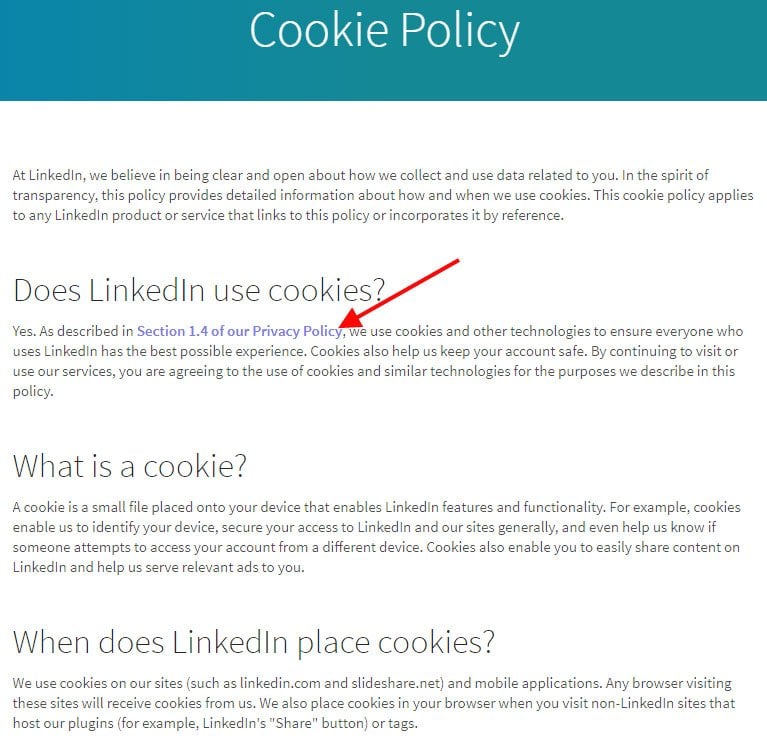**Descriptive Caption for LinkedIn's Cookie Policy Screenshot:**

The image is a screenshot showcasing LinkedIn's cookie policy. At the top of the page, a blue banner prominently displays the title "Cookie Policy." Below the banner, text elaborates LinkedIn’s commitment to transparency in data collection and usage. The policy highlights LinkedIn's use of cookies to enhance user experience and maintain account security, inviting users to agree to these terms by continuing to use LinkedIn services.

A significant mention notes that LinkedIn employs cookies across all their products and services that reference this policy. Specifically, in section 1.4 of the privacy policy, LinkedIn outlines the utilization of cookies and other technologies for an optimal user experience. An added red arrow points directly at the word "policy," drawing attention to this specific document.

Further details explain what a cookie is—a small file placed on the user's device to facilitate LinkedIn's features and functionalities, such as device identification, account security, and content sharing. The text also describes circumstances under which LinkedIn places cookies, not only on its own sites like LinkedIn.com and SlideShare.net but also on non-LinkedIn sites hosting LinkedIn plugins, such as share buttons or tags.

Overall, this detailed cookie policy ensures that users are well-informed about LinkedIn's data collection practices, emphasizing security and user convenience.